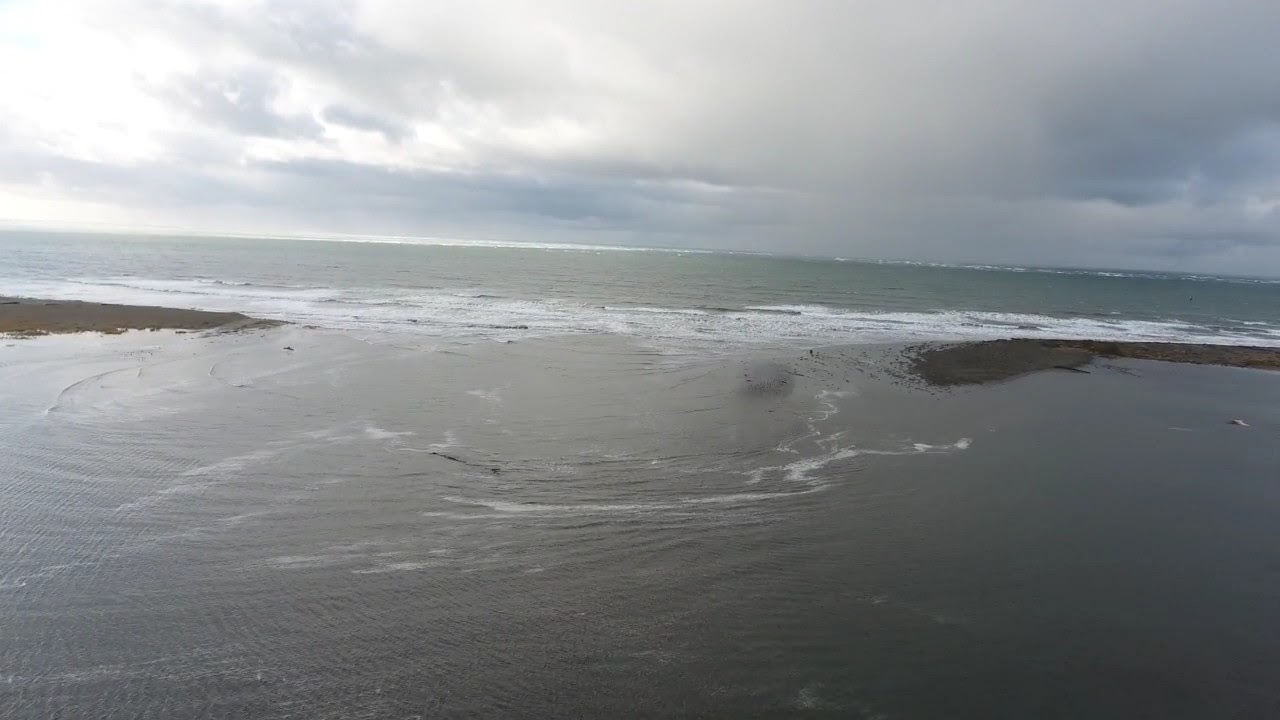This color photograph, captured by a drone in landscape orientation, offers a dramatic and detailed view of a turbulent ocean scene. The vantage point from above provides a sweeping perspective over the greenish dark water, which stretches out to a distant, overcast horizon. Dominating the upper two-thirds of the image, the sky is thick with dark gray clouds, suggesting a rainstorm brewing towards the right-center of the frame. 

In the foreground, waves clash against a sand-covered shoreline that almost resembles a levee, with pockets of water breaking through and creating frothy white crests. This dynamic action of the waves overtopping the sandbars highlights the rough, stormy conditions that might be associated with high tide or even a hurricane. Subtle embankments on the left and right are partially submerged, reinforcing the sense of powerful, relentless water. Meanwhile, in the water, there seems to be an indistinct shape that adds an element of mystery to the otherwise realistic and representational seascape.